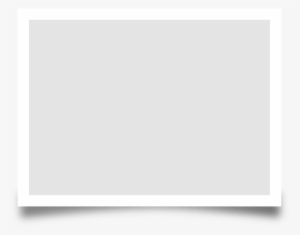This screenshot features a graphical layout that appears to be part of an application interface, though it's unclear whether it is from a mobile app or a desktop application. The composition consists of three nested rectangles, each differing slightly in size and color. The outermost rectangle is light gray and serves as the backdrop for the inner elements. Nested within this is a predominantly white rectangular area, which is slightly smaller and sits centrally within the light gray background. The innermost rectangle, which is dark gray, rests within the white rectangle. 

Interestingly, the white and dark gray rectangles give the illusion of being a single sheet of paper with a slight curvature. This effect is achieved through faint shadows cast at the bottom left and bottom right corners, making it appear as though these corners are lifted slightly off a flat surface, adding a subtle three-dimensional quality to the design.